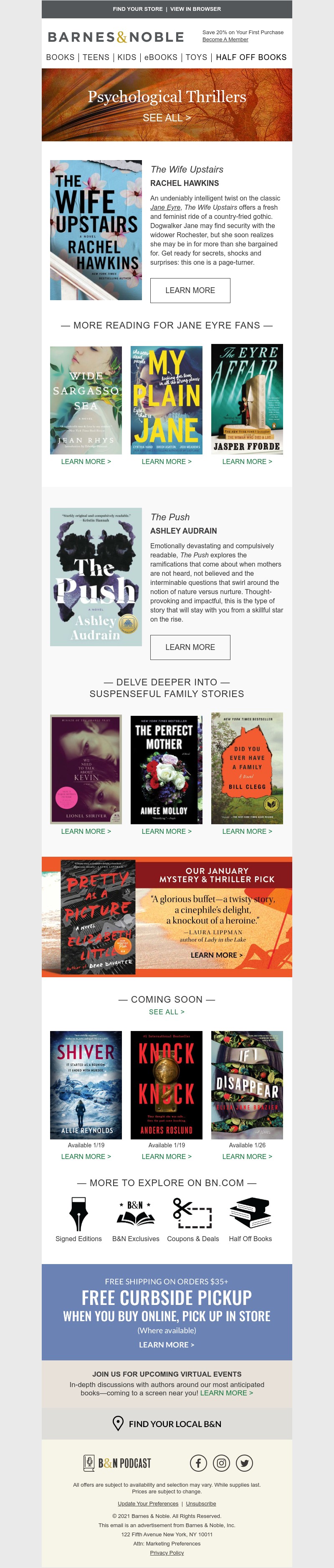A promotional section on the Barnes & Noble website features an eye-catching banner with gold lettering announcing "Psychological Thrillers." Prominently displayed is "The Wife Upstairs" by Rachel Hawkins, accompanied by a detailed description and an invitation to "Learn More." Alongside, three other books are highlighted, further delving into the psychological thriller genre.

Another featured title is "The Push" by Ashley Audrain, with its own description and a "Learn More" option. Following this, three additional psychological thrillers are showcased under a "Coming Soon" section, including "Shiver," "Knock-Knock," and "Disappear."

At the bottom of the section, there is a friendly reminder reading "See Y'all," and a notification about the availability of free curbside pickup, ensuring a convenient shopping experience for customers.